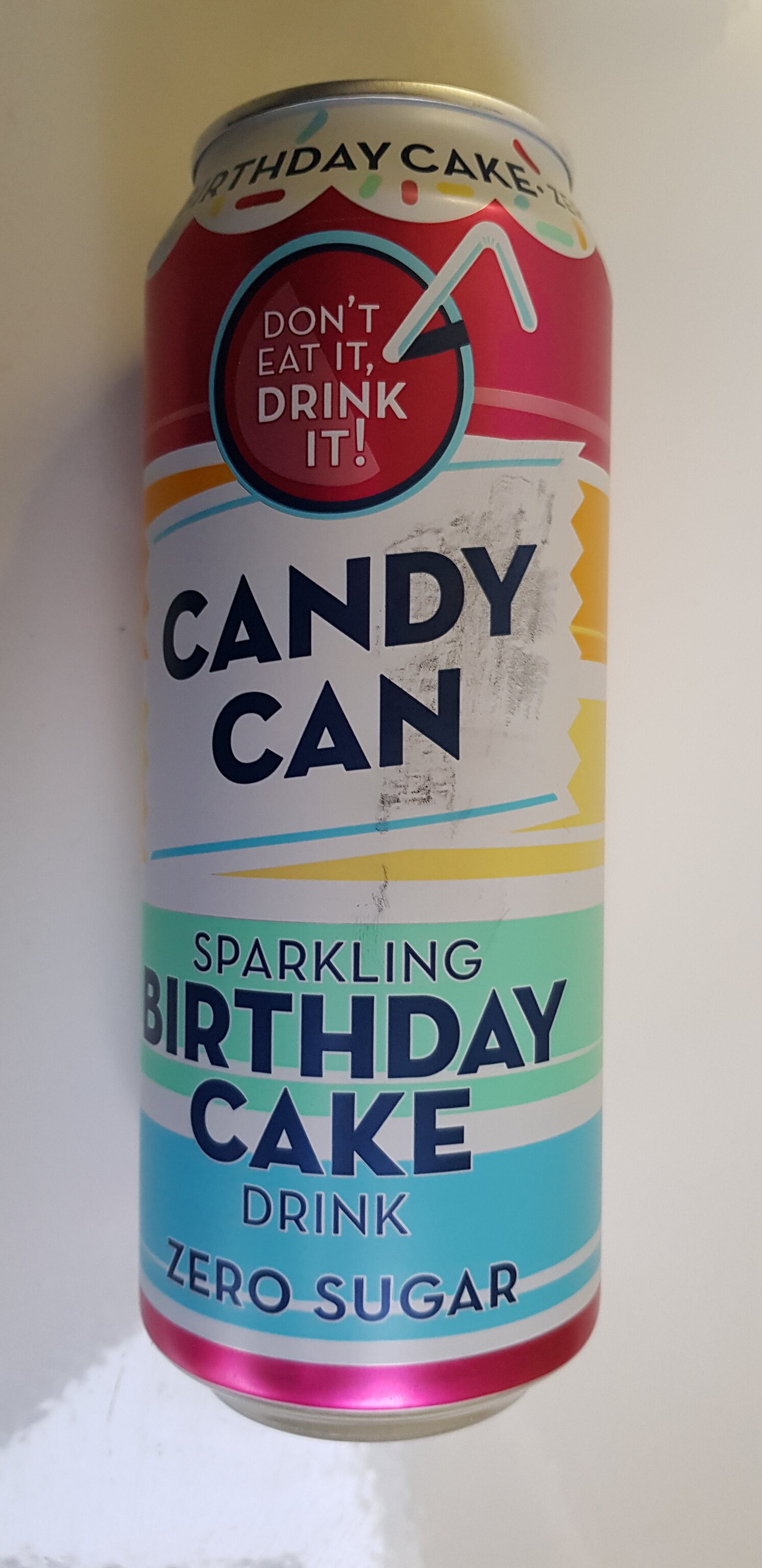The image showcases a tall, thin can labeled "Candy Can Sparkling Birthday Cake Drink Zero Sugar." The can's design is vibrant, featuring a mix of colorful stripes with a pink top and bottom. At the top of the can, just below a scalloped edge, it prominently reads "Birthday Cake" in a bold red font. Beneath this, a circular red icon with a straw sticking out bears the words "Don't eat it, drink it" in white. The central part of the can displays "Candy Can" in a blue font on a white banner, which appears slightly dirty around some letters. Surrounding this banner are horizontal yellow stripes, set against a mint green background that continues with alternating bands of white and blue. The very bottom edge features a thin rose-colored stripe. This detailed and festive design includes additional colors such as green, blue, and yellow confetti, enhancing the celebratory birthday cake theme.